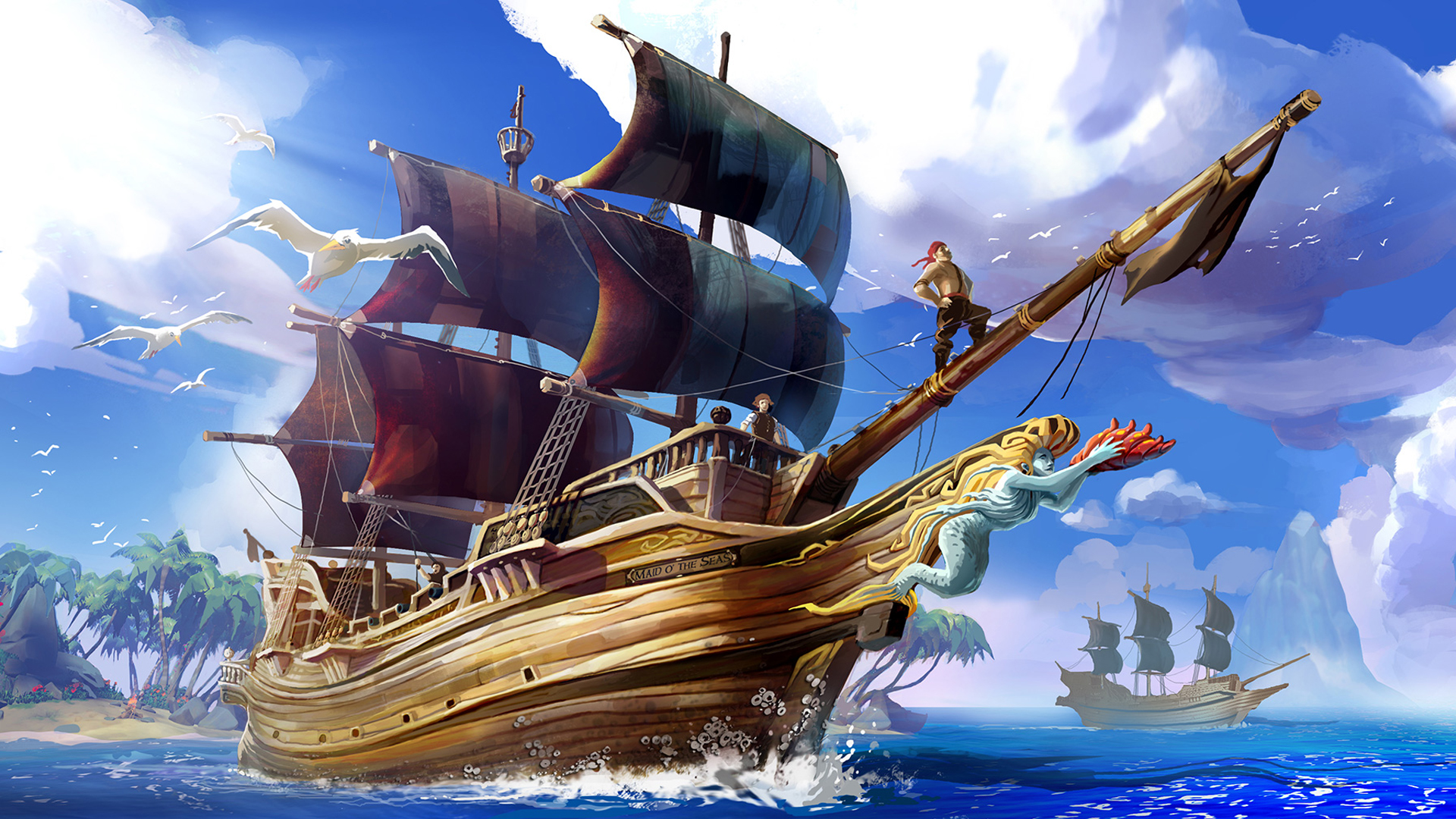The image depicts a detailed and vibrant graphic art poster of a large wooden pirate ship sailing under a clear, blue sky filled with white, fluffy clouds. The ship, sailing towards the right side of the image, is under full sail with three masts, each equipped with dark-colored sails and multiple flags. At the prow of the ship is an intricately carved blue mermaid figurehead with long flowing blonde hair, holding a bright red conch shell.

Several seagulls are depicted flying around the ship, with one particularly close, showing detailed gray wings and orange feet. The ship has multiple decks, portholes, and a crow’s nest on the middle mast where a pirate, donning a red bandana, stands watch, hands on hips, looking out to sea.

In the background, a picturesque island with palm trees and a sandy beach stretches out, indicating where the ship has recently departed. Another similarly designed pirate ship with three masts is seen in the distance, moving across the calm sea decorated with gentle white waves, suggesting its motion through the water. The overall scene is dreamlike, combining elements of classic pirate lore with fantastical details. The name of the main ship is likely "Maid of the Seas," adding an additional layer of mystique to this captivating maritime artwork.